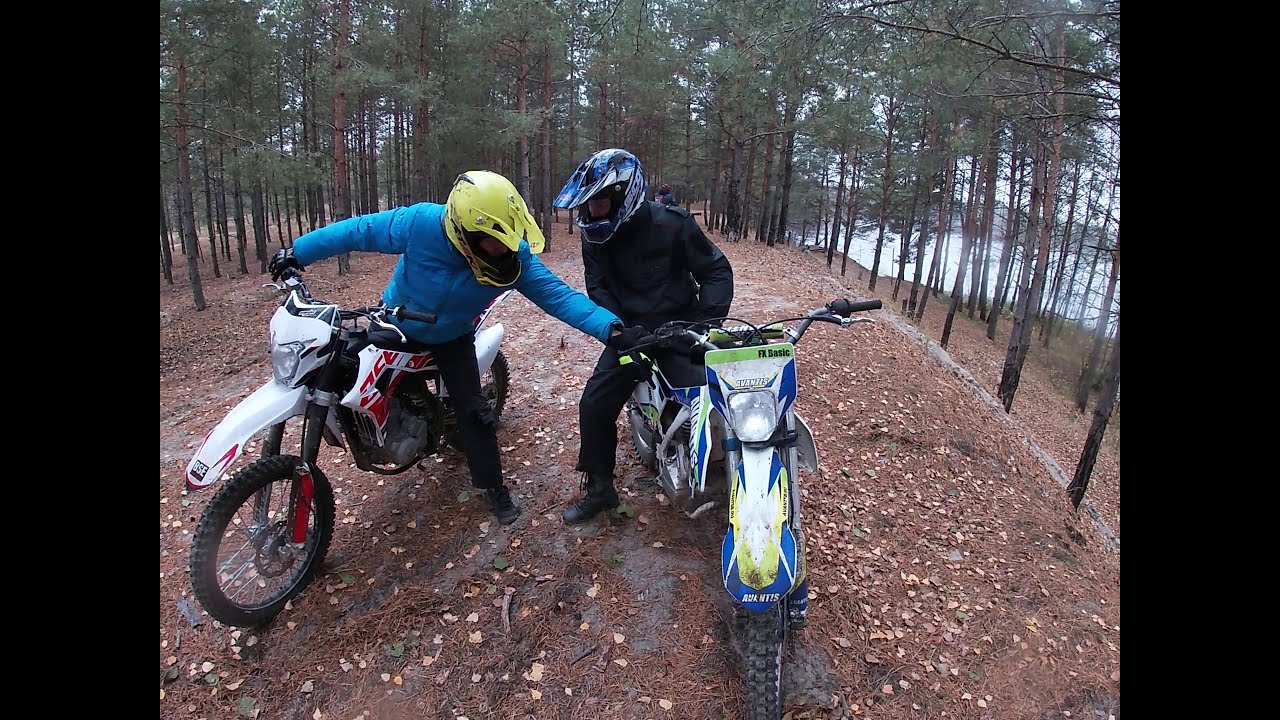In a forest clearing covered with brown, leaf-strewn dirt, two men are paused on their dirt bikes, closely examining each other's bikes. The man on the left, wearing a bright blue jacket, black pants, and a greenish-yellow helmet, is reaching out toward the other rider's handlebars. His red and silver dirt bike is angled towards the 7 o'clock position, and he has his left foot planted on the ground. The other man, in a dark outfit with dark shoes and a blue and white helmet, stands next to his dirt bike, which faces directly at the camera. This bike is blue, yellow, silver, and green. He supports himself with both feet off his bike, looking toward his companion. In the background, tall, slender trees flank the scene, and a glimpse of water can be seen through their trunks under the clear daylight. The ground is entirely covered in dead leaves, adding to the natural, forested atmosphere.